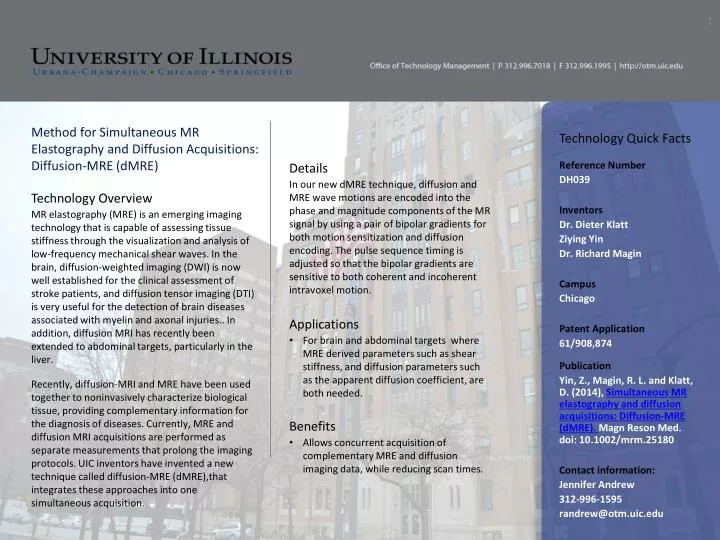Screenshot of the University of Illinois website. Across the top, there is a dark gray navigation bar featuring black text on the left-hand side. The first line states "University of Illinois." Below that, in small blue lettering, it mentions something related to a "campaign," followed by the word "Chicago" and additional blurry text. On the right of these lines, in very small white text, it reads "Office of Technology Management," along with what appears to be a phone number and a website. 

Below the navigation bar, the main content is divided into three columns. The first two columns on the left have a white background adorned with a faint image, likely of the college campus. Overlaying this imagery is some form of explanatory or descriptive text, possibly detailing the content or purpose of the website. The third column on the right is colored blue and contains concise "quick facts," which seem to summarize the key information presented on the website.